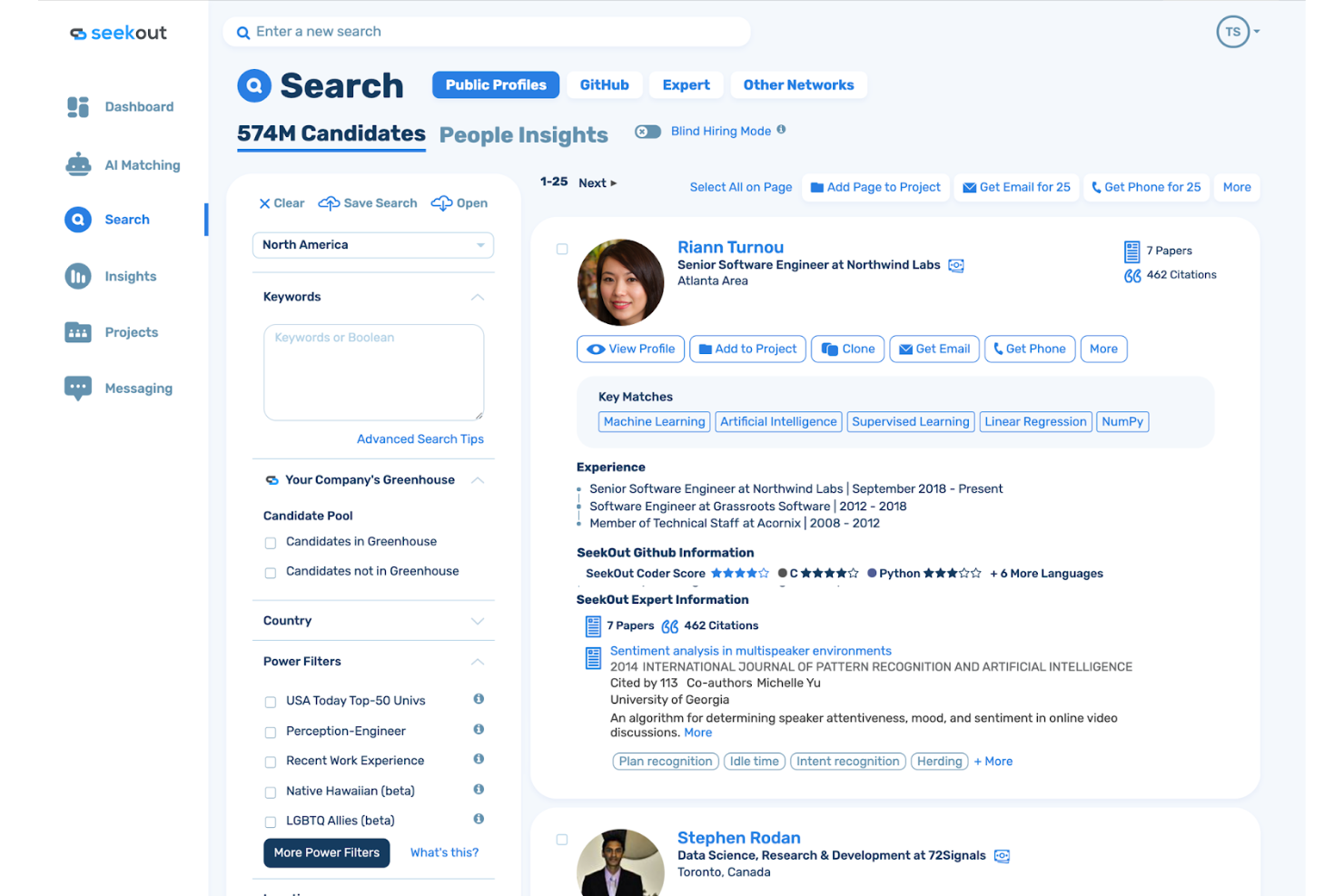**Caption:**

This image shows a digital interface from the website SeekOut, designed for recruiting and accessing professional credentials. The website's name, "SeekOut," is prominently displayed with "Seek" in light blue and "Out" in dark blue, combined into a single word. On the left side of the interface, there is a white tab or sidebar featuring multiple options in a grayish-blue tone. These options include Dashboard, All Matching, Search (currently selected and highlighted in dark blue), Insights, Projects, and Messaging.

The main screen on the right allows users to enter a new search at the top. Just below that, there is an icon of a magnifying glass next to the word "Search" in large, bold letters. Users can search through various sections like Public Profiles, GitHub, Expert, and Other Networks, with Public Profiles currently selected, indicating 574 million candidates available. Adjacent to this section is "People Insights."

Visible user profiles are part of the search results. One featured profile is of Rhianne Turnow, a Senior Software Engineer at Northwind Labs based in the Atlanta area, who appears to be of Asian descent. Options to view her profile and contact her are available. Another profile shows Steven Rodin, a dark-skinned gentleman who is involved in Data Science Research and Development at Seventy Signals, located in Toronto, Canada.